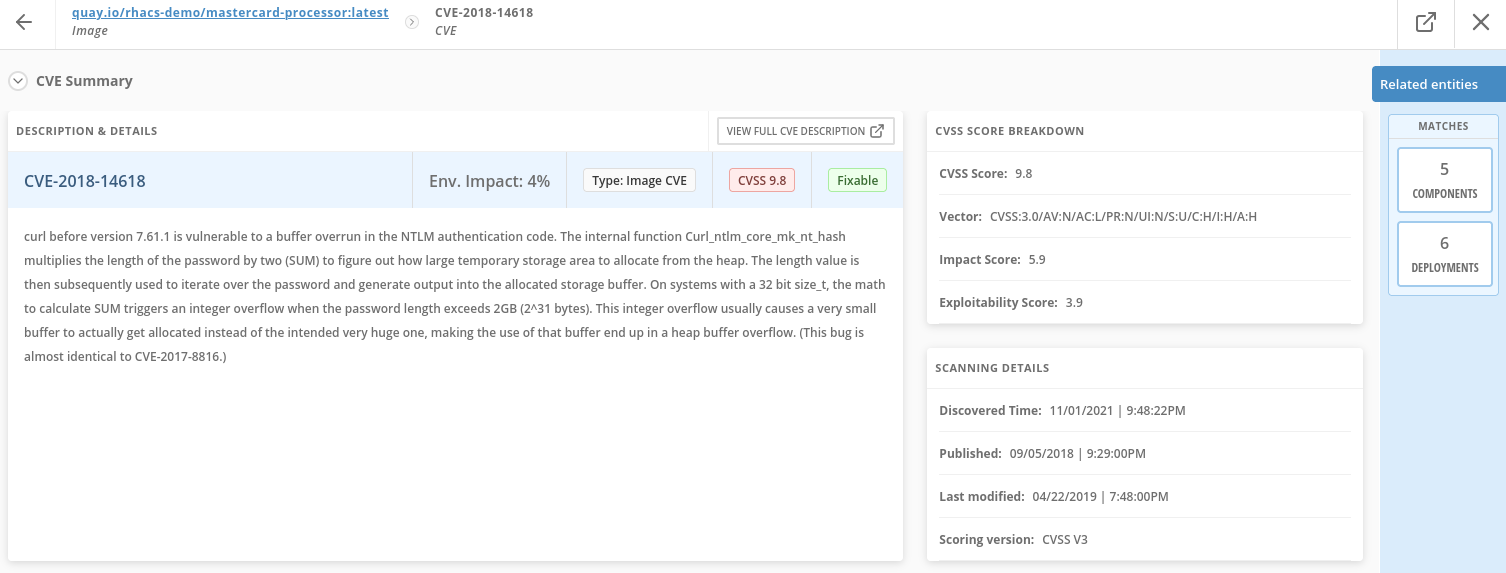**Detailed Caption for the Image:**

The image depicts a detailed screenshot of a webpage displaying a CVE (Common Vulnerabilities and Exposures) Summary, specifically for CVE-2018-14618. 

**Header Section:**
- At the top left corner of the page, there is a back arrow symbol, suggesting a navigation option to return to the previous page.
- Adjacent to the back arrow is a hyperlink titled "quay.io/RHACS-demos/mastercard-processor:latest." 
- Following the hyperlink, a forward arrow is shown with the label "CVE-2018-14618."

**Content Section:**

**CVE Summary:**
1. **Description and Details:**
   - CVE ID: CVE-2018-14618
   - Environmental Impact: 4%
   - Type: Image
   - CVSS Score: 9.8 out of 10.
2. There is a green button labeled "Fixable," indicating that a solution to the vulnerability exists.

**Main Text:**
- The description details a vulnerability in Curl before version 7.61.1, specifically a buffer overrun issue in NTLM authentication code.
- The internal function `curl_ntlm_core_mk_nt_hash` multiplies the password length by two (referred to as SUM) to ascertain the temporary storage area size to allocate from the heap.
- For systems with a 32-bit size_t, if the password length exceeds 2GB (2^31 bytes), an integer overflow occurs during the calculation.
- This overflow results in a considerably smaller buffer being allocated instead of the expected large buffer, leading to a heap buffer overflow.
- The bug presents similarities to a previous issue identified as CVE-2017-8816.

This caption summarizes the information comprehensively and elucidates the context of the CVE summary detailed in the image.